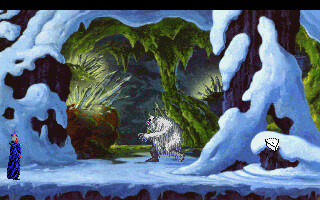The illustration appears to be a vibrant and colorful scene, likely from a video game or animated cartoon, depicting a snowy, cavernous environment. The focal point is a monstrous figure resembling a yeti, with thick white fur, outstretched arms, and a forward-stepping leg, implying movement towards a specific target. This target seems to be a human-like figure, dressed in a long, dark blue robe, possibly a wizard, situated to the left of the yeti. The cave setting is rich in detail, with a snowy exterior leading into an interior that is lush with green moss and long, green crystals, adding a mystical quality to the scene.

The background showcases a winter landscape with snow-covered trees on both sides, framing the entrance to the cave. The snowy surroundings extend into the foreground, where rocks too are blanketed in snow. Amidst this setting, light can be seen emanating from the cave's deeper recesses, creating a pathway of illumination that enhances the scene's depth and atmosphere. The depiction of the yeti, though small and somewhat indistinct, suggests a creature more ghostly or possibly frozen, adding an eerie element to the image.

Overall, this detailed scene pulls the viewer in with its elaborate wintery landscape, fantastical cave interior, and intriguing characters, suggesting a narrative filled with magic and suspense.